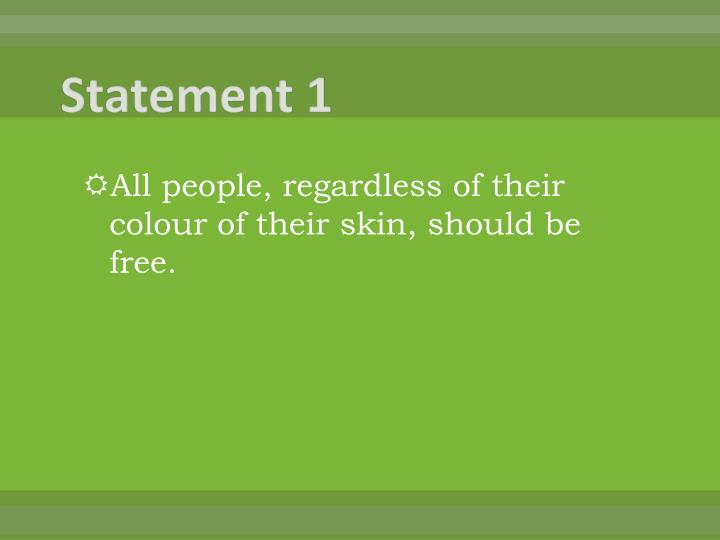The image appears to be a PowerPoint slide that is rectangular and slightly wider than it is tall. It presents text against a layered green background. At the top, there is a band of dark olive green, followed by a narrow strip of a slightly muted green. Below this is another wider band of olive green which contains the title "Statement 1" in white letters on the upper left corner of the slide. The middle section of the slide has a large lime green area where the main content is displayed. The main text, also in white letters, reads: "All people, regardless of their color of their skin, should be free." This middle portion of the slide contains the text in three lines, with an outline of a sun next to the first line. Lastly, the bottom part of the slide features a narrow darker green band, maintaining a consistent color variation to create texture for the presentation.